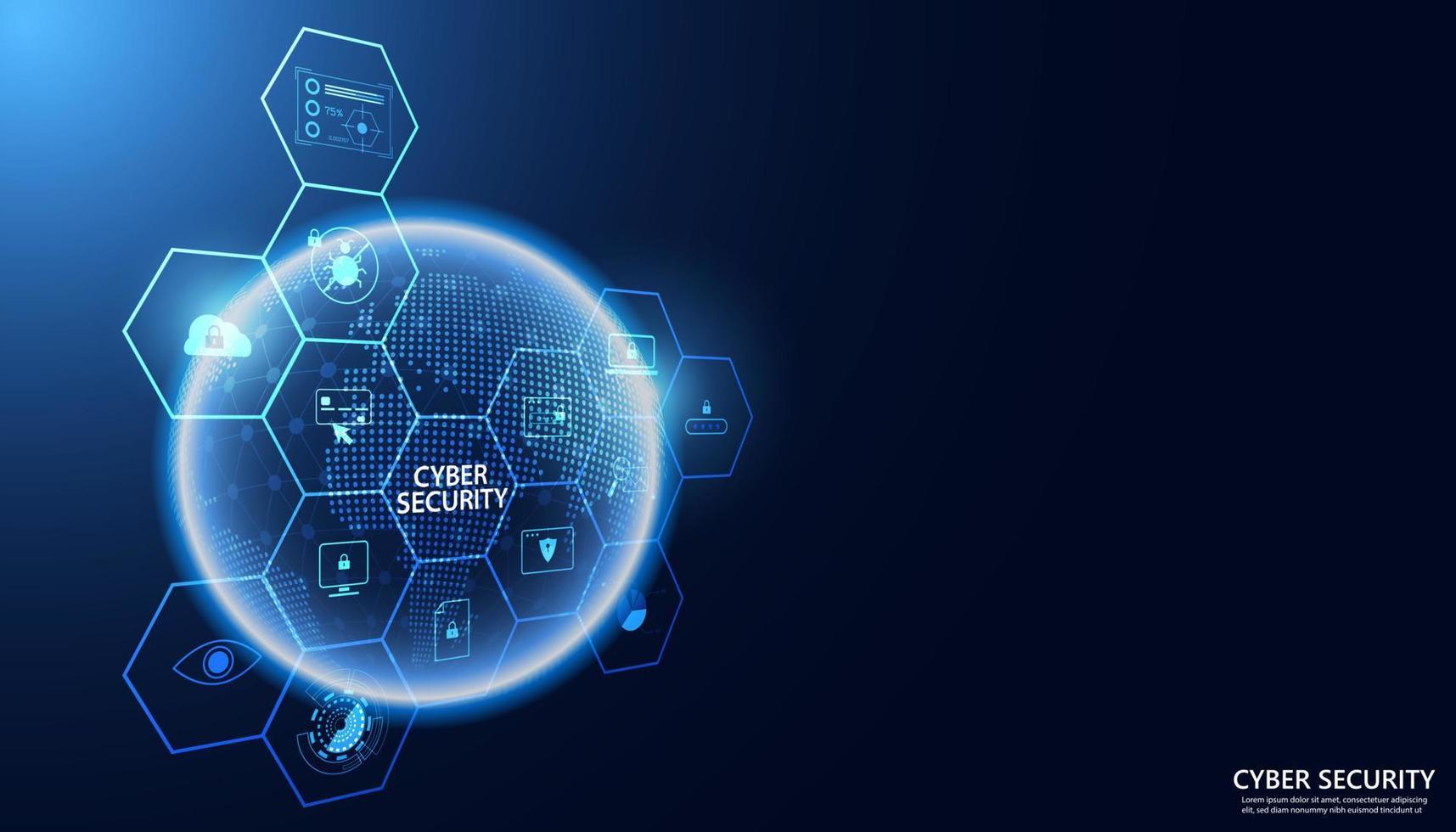The image features a predominantly dark blue background, with the right side being solidly dark blue except for the bottom right corner where the white text "Cyber Security" is displayed, accompanied by smaller, illegible white text beneath it. The left side of the image is dominated by a techno blue glowing sphere, resembling the Earth, adorned with numerous small square dots outlining the continents. Overlapping the sphere is a honeycomb pattern of neon light blue hexagons. Each hexagon contains an individual image in a similar light blue color; notable among them are icons of computer monitors with locks, a shield, a cloud with a lock, an eyeball, an insect with an 'X' through it, a padlock, a pie chart, and a location symbol. Centrally placed within one of the hexagons is the text "Cyber Security." The overall composition suggests a promotional graphic, possibly illustrating the comprehensive scope of a cyber security firm's services, akin to a business card without specific contact details.